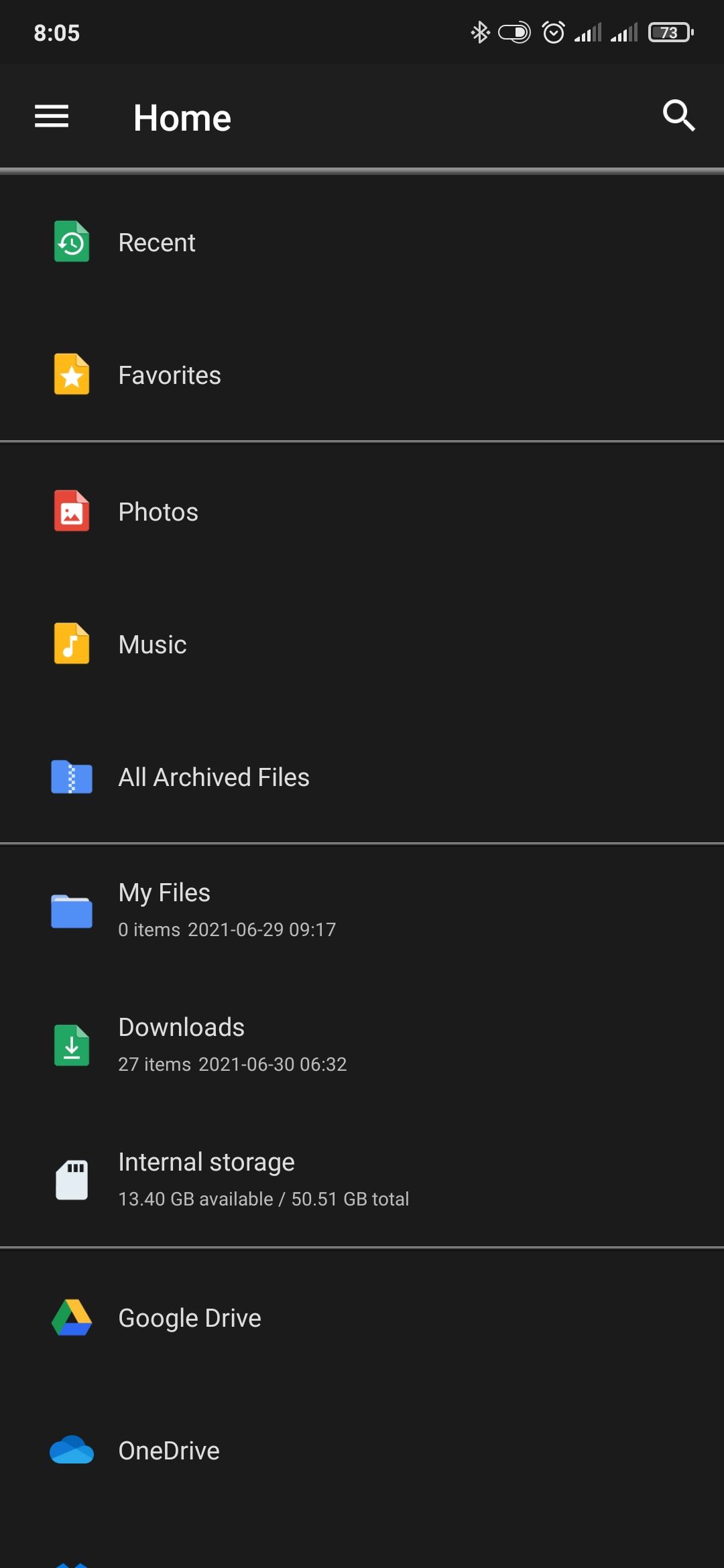A screenshot displays a phone settings screen with a dark theme enabled, giving it a black background. The time "8:05" is visible in the top left corner, while the battery indicator shows approximately two-thirds charge. On the right side, Bluetooth is turned on, and there's an additional battery icon showing 73% charge. An active alarm, represented by an icon, is also visible. Both Wi-Fi signals have three bands.

Beneath these icons, on the left side, there are three horizontal lines indicating a menu button. To the right of it, the word "Home" is displayed prominently in large white letters, with a white magnifying glass icon for search functionality located on the far right. 

The main section contains several icons and labels arranged vertically. Starting at the top left, there's a green icon followed by the text "Recent" in white. Below it is a yellow icon with a white star next to the word "Favorites." 

Continuing downward, a red icon with a white square labeled "Photos" is followed by an orange folder icon with a white music note labeled "Music." Next is an icon depicting a file folder with a zigzag white line down the center, labeled "All Archive Files." Subsequently, a standard file folder icon labeled "My Files" is visible.

Further down, a green icon with a white downward arrow appears, labeled "Downloads." Below this, a white folder icon marked "Internal Storage" is shown. Finally, a multicolored triangle icon representing Google Drive is labeled accordingly, and beneath that is a two-tone blue cloud icon with the label "OneDrive."